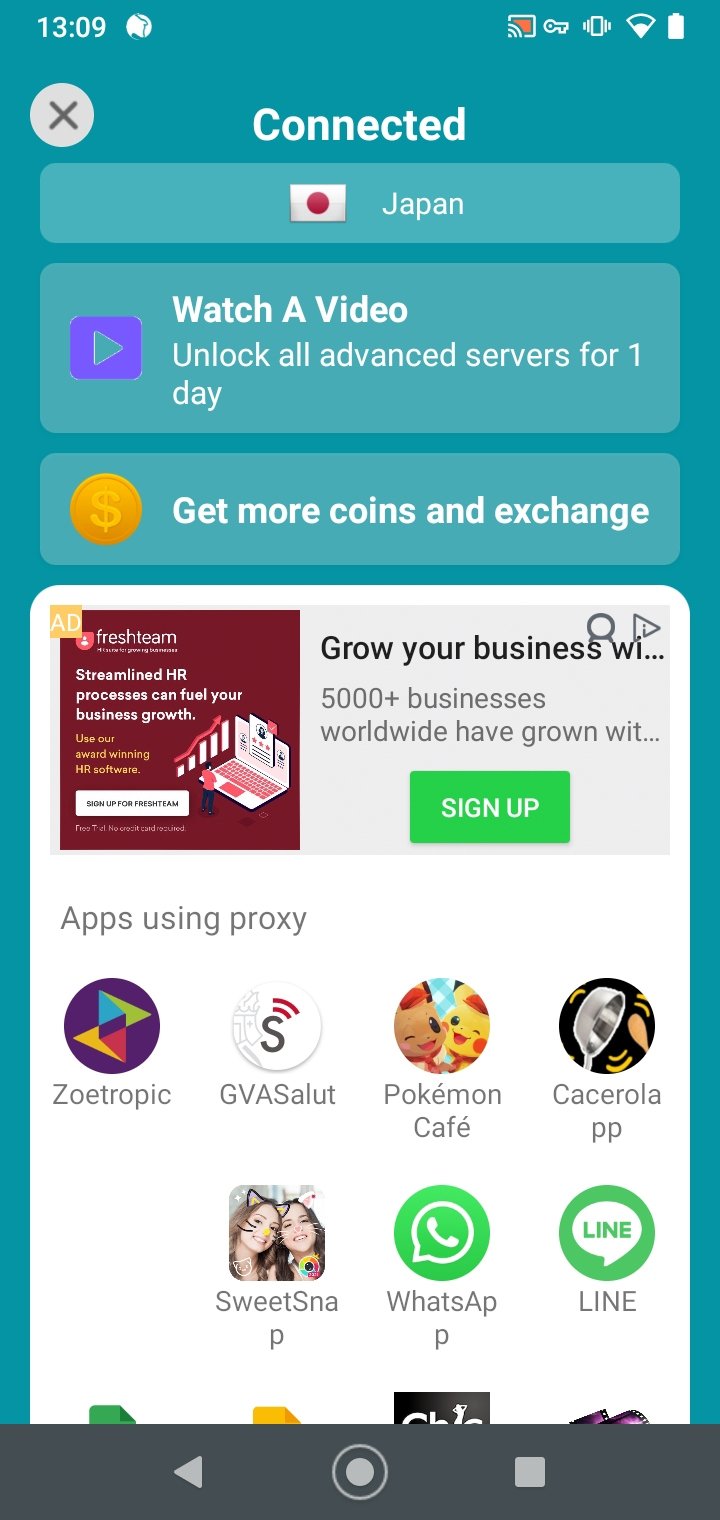The image displays a mobile device, possibly a phone or tablet, running an application. In the upper left-hand corner, the time is shown as 13:09 in white. In the upper right-hand corner, there are icons indicating Wi-Fi casting, a key (possibly denoting secured connection), vibration mode, and a fully charged battery. Below these icons, a gray square with a black X, and the word "connected" written in white, suggests an option to close the connection status.

The background features a teal blue color with slightly lighter blue windows or sections. One of these windows displays "Japan" with a Japanese flag. Other sections promote in-app opportunities, such as "Watch a video, unlock all advanced servers for one day" with a purple icon, and "Get more coins in exchange" accompanied by a gold coin icon. 

An advertisement for Fresh Team is prominently featured, promoting streamlined HR processes for business growth. It mentions, "Use your award-winning HR software, grow your business. 5000+ businesses worldwide have grown" and includes a "Sign Up" button.

At the bottom, a list of apps using proxy services is displayed, including Zeotropic, GVA Salute, Pokémon Café, Casserole PP, Sweetsnap, WhatsApp, and Line.